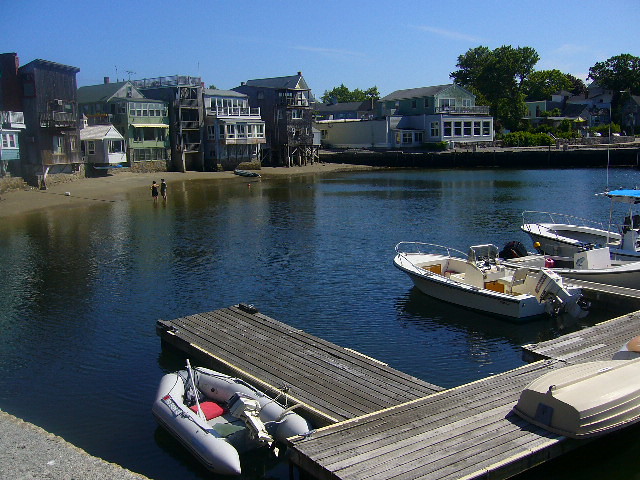The photograph captures a vibrant outdoor scene on a bright, sunny day with a mostly clear, blue sky dotted by a few wisps of clouds. In the background, tall trees frame several houses—some of them large and likely summer homes, while others are smaller. These homes line a calm lake, creating a peaceful shoreline backdrop.

In the lake's shallow waters stand two people, facing the homes. Nearby, a collection of boats are tied to a wooden dock. This includes three small boats equipped with outboard motors, one of which features a blue roof. Additionally, there is a small inflatable raft with a motor and an upside-down rowboat resting on the dock. At the lower left of the image, a stone walkway leads to the dock, completing this tranquil lakeside setting.